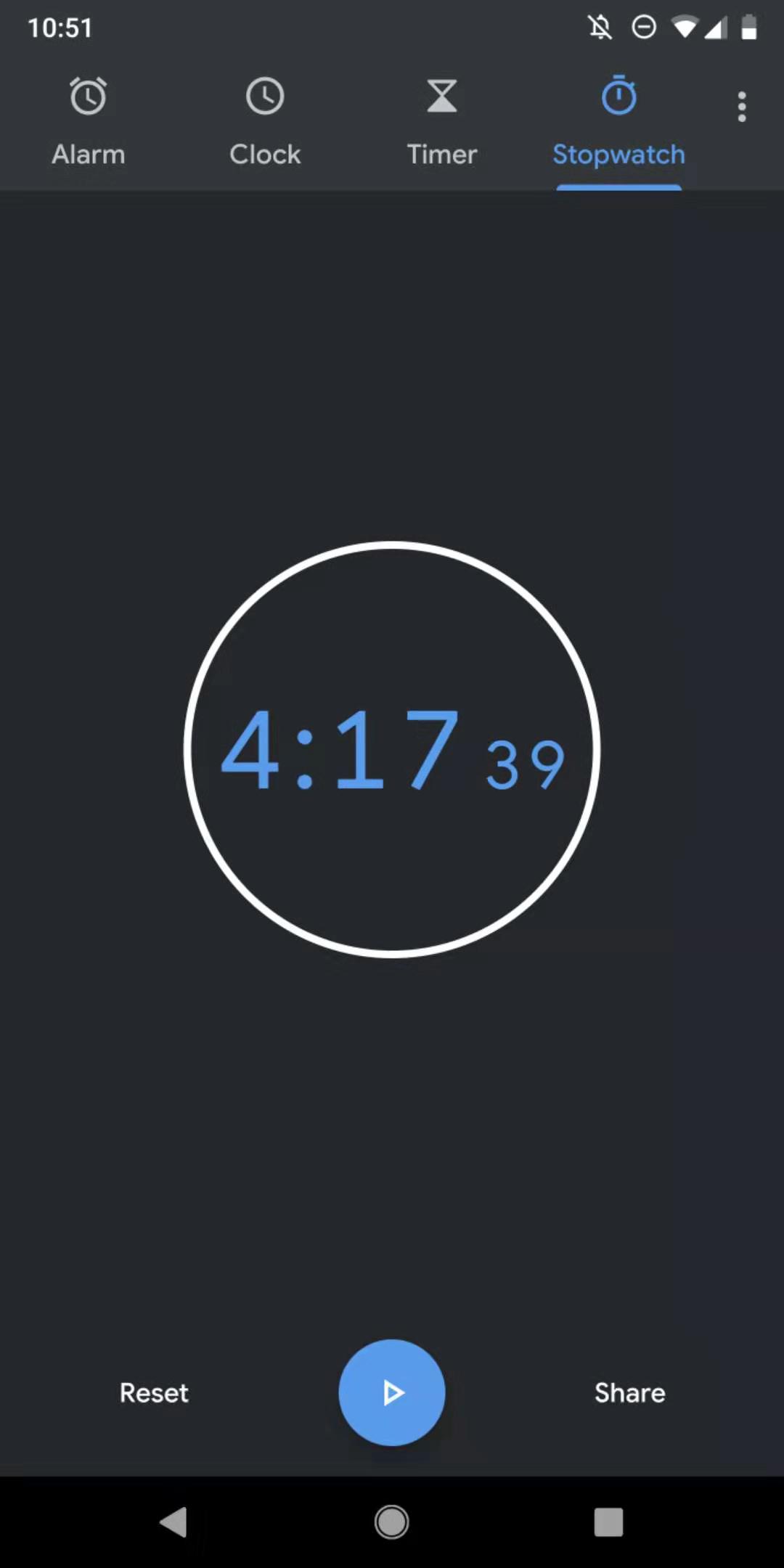This image is a clear screenshot from a cell phone, focusing on the stopwatch function. The background is predominantly black, with the upper banner slightly lighter black to create a contrast. In the upper left corner, the time is displayed in white font as "10:51." The upper right corner features five icons pertaining to cell phone statuses such as battery life, signal reception, and the alarm status, which appears to be off. 

Near the top of the screen, there are four selectable menu items: "Alarm," "Clock," "Timer," and "Stopwatch," with "Stopwatch" highlighted in blue. This selection is further emphasized by a blue underline. Additionally, three vertical white dots are displayed in the upper right corner, indicating more menu options.

The center of the screen prominently displays the stopwatch in action, with the digits "4:17" in white font and smaller blue digits "39," representing either four minutes, seventeen seconds, and thirty-nine hundredths of a second, or potentially four hours, seventeen minutes, and thirty-nine seconds.

Beneath the main display, two options are visible in white font: "Reset" on the left, and "Share" on the right. At the bottom of the screen, a blue circle containing a white triangle points to the right, indicating the play button, flanked by symbols for recording and navigating back.